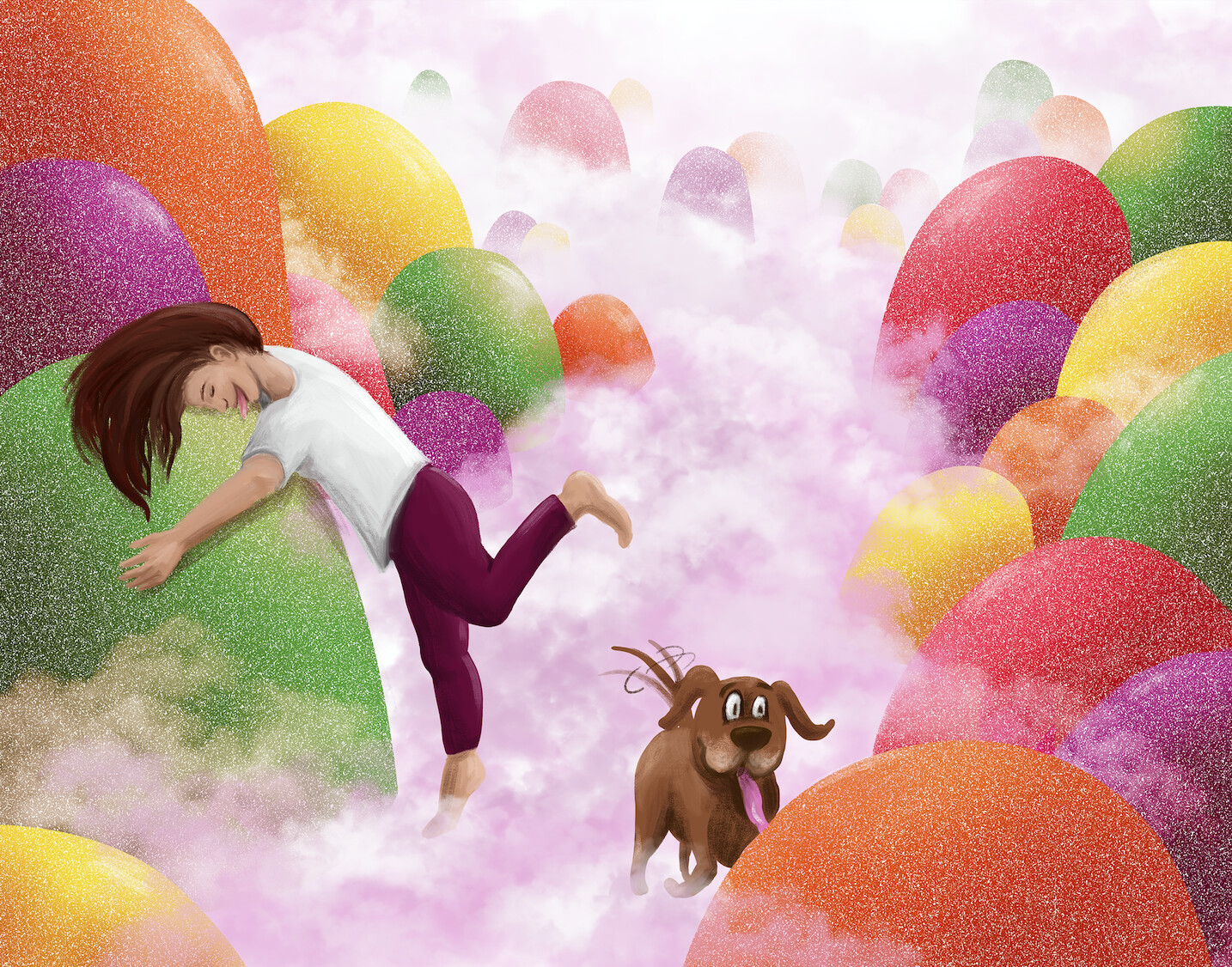The illustration depicts a whimsical scene filled with colorful, egg-shaped or gumdrop-like objects in various hues, including green, yellow, orange, red, and purple. These vibrant objects are scattered across the background and both sides of the image, some even dusted with what looks like powdered sugar. Central to the scene is a mist of fluffy pink and white clouds.

On the left side of the image, a young girl with long brown hair is hugging a large green egg-shaped object. She is wearing a white t-shirt and maroon leggings. With her face pressed against the top of the object, she playfully sticks out her tongue. Her pose is dynamic, with one leg extended and bent behind her, her foot in the air, and the other leg tiptoeing.

To her right, a cheerful brown cartoon dog faces the viewer. The dog has expressive tall white eyes with black pupils, long ears that curl at the ends, and a pink tongue sticking out. Its tail wags vigorously, indicated by black motion lines, and its legs are positioned as if in mid-movement, conveying a lively playfulness. The entire scene is infused with a sense of fun and whimsy, typical of a delightful cartoon world.